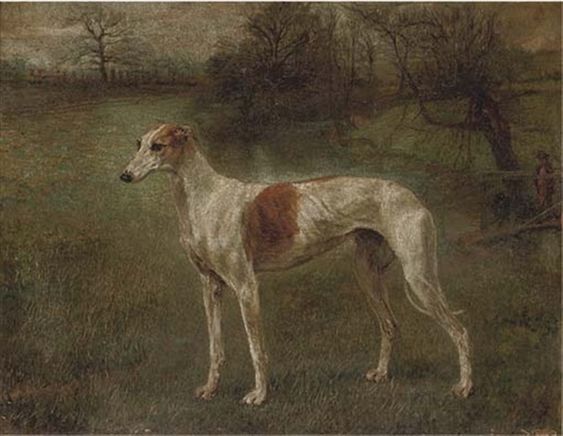This painting, rectangle in shape, features a tall, slender greyhound dog prominently positioned in the center, looking towards the left. The dog has a distinctive appearance with a predominantly white coat, accented by a large brown spot on its torso and another brown marking extending from its left eye, over its ear, and down to its neck. The greyhound's thin, white tail is tucked between its legs, and its ribcage is visibly outlined. The background is a somber blend of brown and gray, suggestive of a dreary, cold month, likely winter. This older painting exudes an 1800s aesthetic, with dead trees dotting the upper right and a mix of brown and green grass in the foreground. A small stream can be seen in the distance, with a man, and possibly a child, standing near a bridge on the right side. The overall scene suggests a desolate field, emphasizing the elegant, poised figure of the greyhound amidst a stark and wintry landscape.